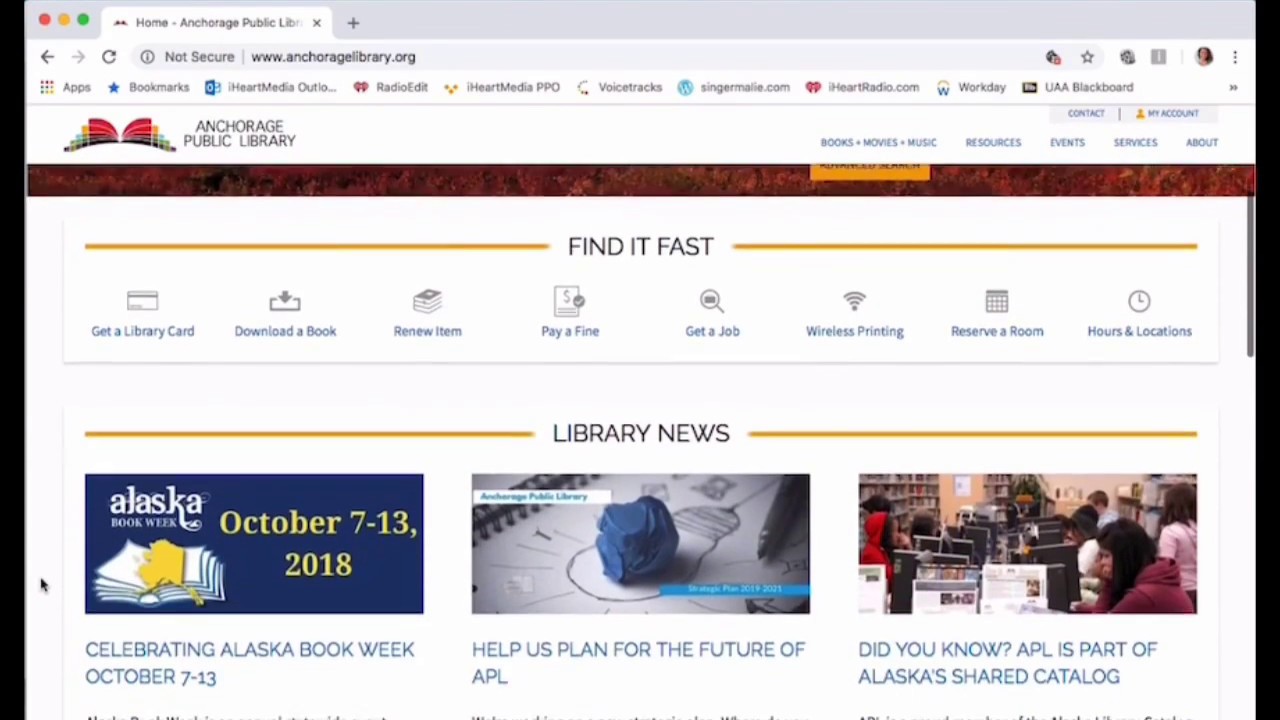This image captures a busy scene at the Anchorage Public Library, prominently showcasing the banner celebrating Alaska Book Week, held on October 7th, 2013. The banner encourages patrons to help plan for the future of the library, emphasizing the library's role in the Alaska Shared Catalog. A yellow highlight prominently displays a "Find it Fast" section, offering quick access to download books, renew items, pay fines, do wireless printing, reserve meeting rooms, and find library hours and locations.

In the foreground, a rotating selector menu presents various options, including resources such as books, movies, music, events, and services provided by the library. The website AnchorageLibrary.org and various associated media outlets like iHeartMedia are mentioned, showcasing the library’s broad digital integration.

A rock placed on a sketchbook and a hanging lightbulb suggest a creative and thoughtful ambiance, as users engage in study and research. Patrons are seen seated at computers and tables, deeply engrossed in their activities. The background of the image features a warm brown color, enhancing the cozy and inviting atmosphere of the library space.